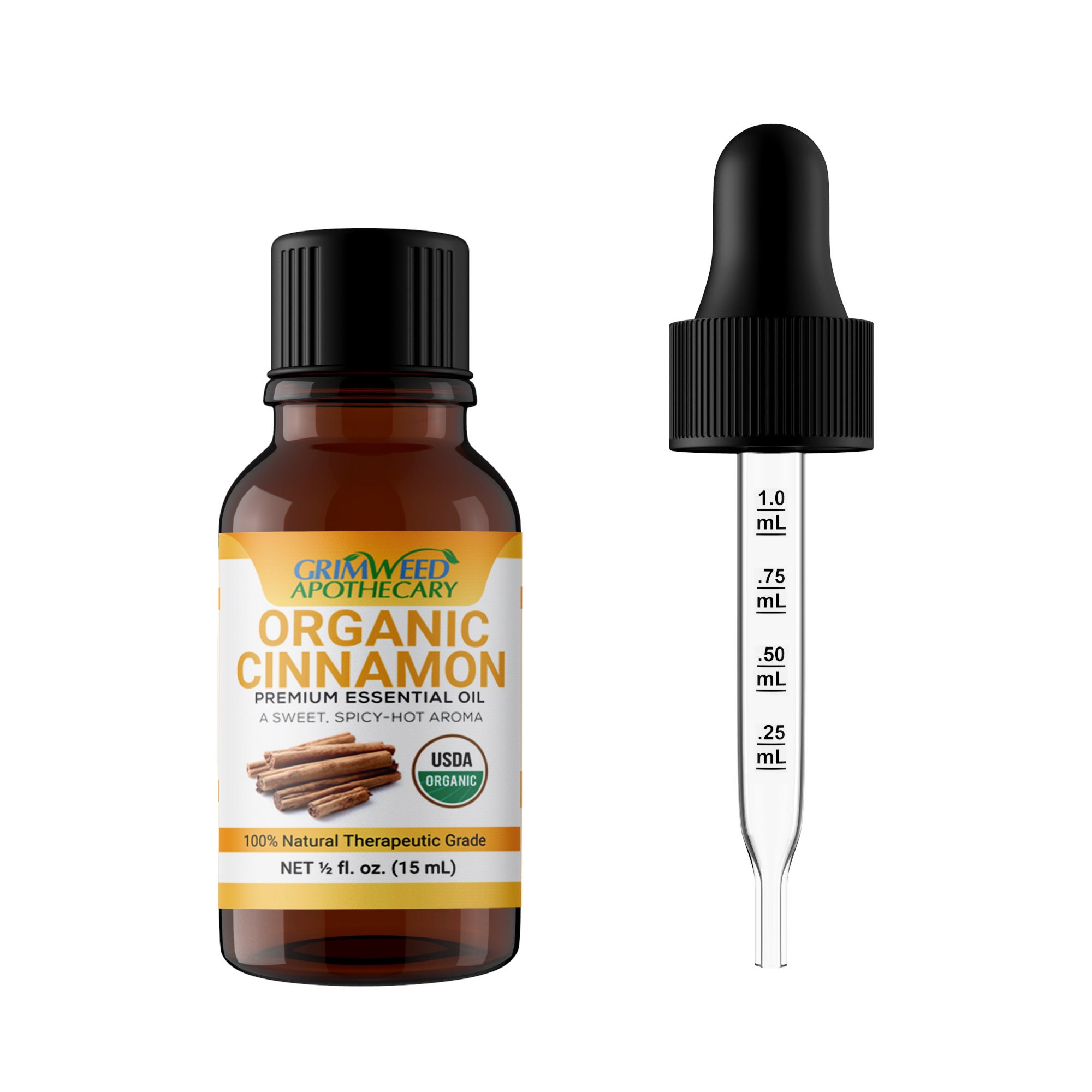This advertisement photo for Grimweed Apothecary showcases a meticulously detailed presentation of their Organic Cinnamon Premium Essential Oil. On the left, the brown glass vial with a black cap displays a comprehensive label featuring the Grimweed Apothecary brand, along with a clear graphic of cinnamon sticks. The label highlights key details: "Organic Cinnamon Premium Essential Oil" in orange font, promising a sweet, spicy, hot aroma, and certifies the product as USDA organic and 100% natural therapeutic grade. The bottle holds a net volume of half a fluid ounce, approximately 15 milliliters. Positioned on the right side is a complementary clear dropper with a black rubber top, marked with measurement lines at 1.0 ml, 0.75 ml, 0.50 ml, and 0.25 ml, ensuring precise dosage of the essential oil. The high-quality image effectively illustrates the product's appeal and functionality, catering to potential buyers.